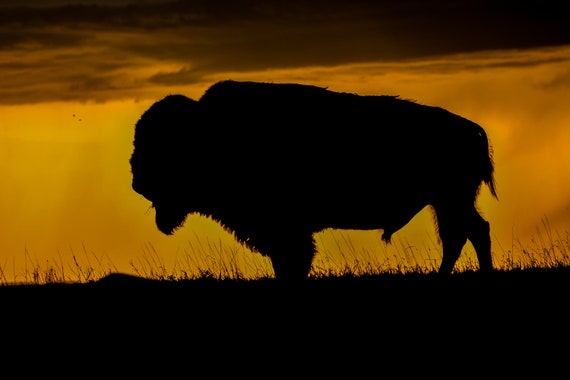This photograph captures a striking silhouette of a buffalo or American bison, centralized in the frame, amidst an evocative landscape. The image showcases a deep black silhouette of the buffalo standing atop a silhouetted grassy terrain. The buffalo’s prominent outline reveals its strong front legs, thinner rear legs, distinct beard, rectangular head, and wispy tail. Unique details such as the tuft of hair around its genital area are also visible. The background is a vibrant gradient of deep orange and yellow hues, possibly indicating a sunset, with dark, ominous clouds featuring an orange underside just above. The composition is divided into three distinct sections: the dark silhouetted ground at the bottom with tufts of grass, the bright orange and yellow middle background sky, and the dark, cloudy sky at the top, merging together to create a visually compelling scene dominated by shades of black and orange.